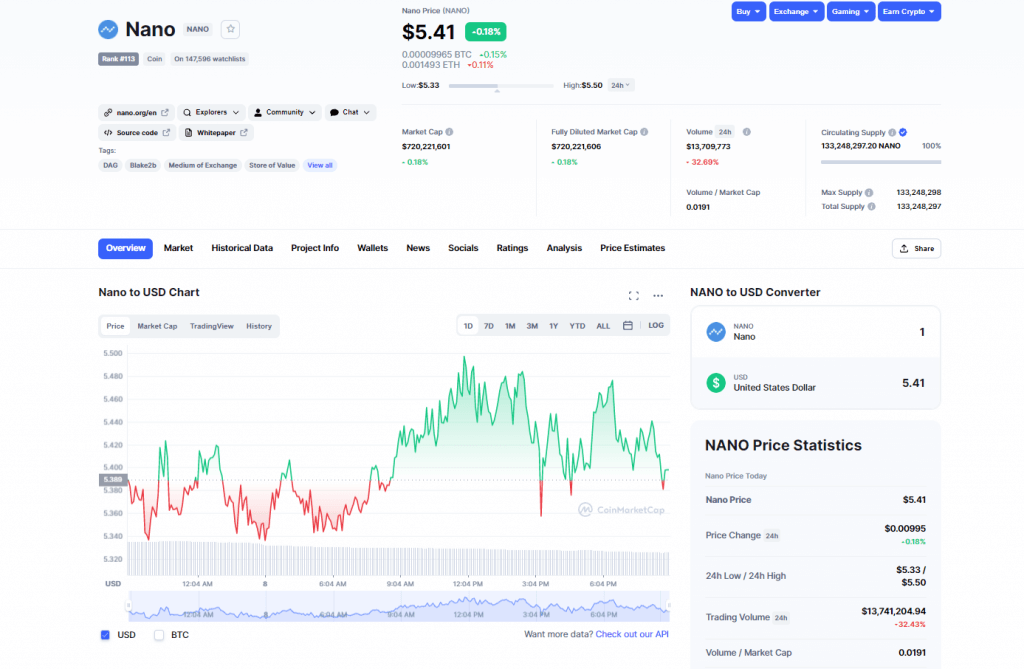The image displays a comprehensive cryptocurrency trading interface, prominently featuring a detailed price chart for Nano (NANO). The top-left corner includes the Nano logo, a blue icon with a squiggly line, and the current Nano price, listed as $5.41. Below the price, it shows equivalent values in Bitcoin (BTC) and Ethereum (ETH). 

The primary feature of the interface is a large, detailed chart tracking Nano's price fluctuations over the day, with time stamps running from 12:04 AM to 6:04 PM. The peaks and valleys indicate how the value of Nano has risen and fallen throughout the day, with the current price being slightly higher than earlier.

The interface follows a clean, modern design with a white background, blue navigation buttons, and black text. In the upper right corner, there are functional buttons labeled "Buy," "Exchange," "Gaming," and "Earn Crypto." These options suggest additional features and services available on this platform beyond simple price tracking.